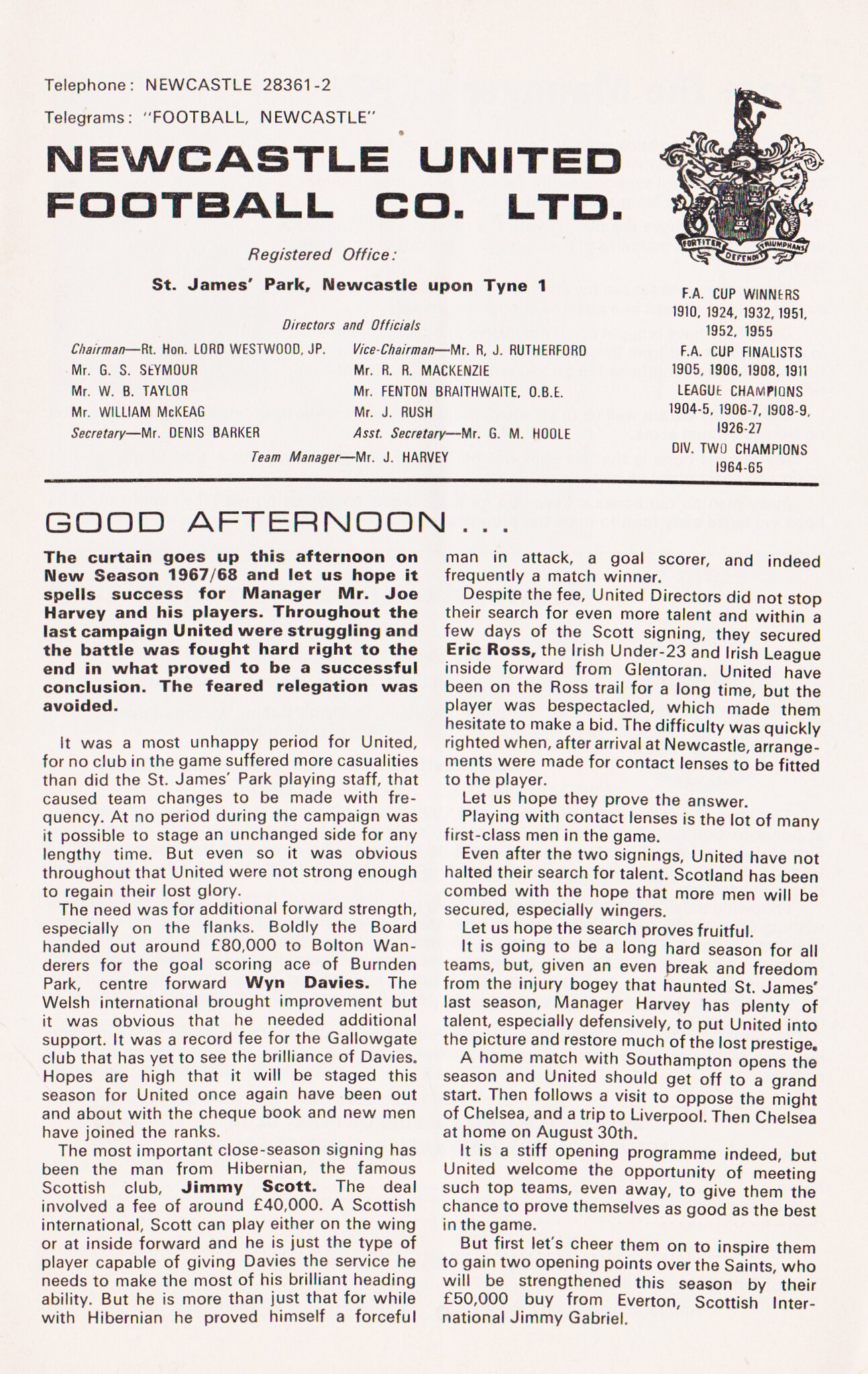The image is a page from an official Newcastle United Football Club program or newsletter, featuring a gray background in the upper left. At the top, it displays the contact information: "Telephone Newcastle 283612" and "Telegrams: Football, Newcastle." Below that, in prominent black font, it states "Newcastle United Football Co. LTD" and to the right of this, there's the club's black and white crest. The text continues with the registered address: "Registered Office: St. James Park, Newcastle upon Tyne 1." Further down, it lists several directors and officials, including Chairman R.T. Hon. Lord Westwood, J.P., Mr. J.S. Seymour, Mr. W.B. Taylor, Mr. William McKeague, and Secretary Mr. Dennis Barker. 

The main body of the page welcomes readers with "Good afternoon..." followed by several paragraphs beginning with, "The curtain goes up this afternoon on new season 1967-68 and let us hope it spells success for manager Mr. Joe Harvey and his players." It goes on to recap the previous challenging season, noting that United struggled but ultimately avoided relegation despite numerous injuries. The header text is separated from the body by a line, and a banner with the motto "48 Defended Triumphant" appears beneath the crest.